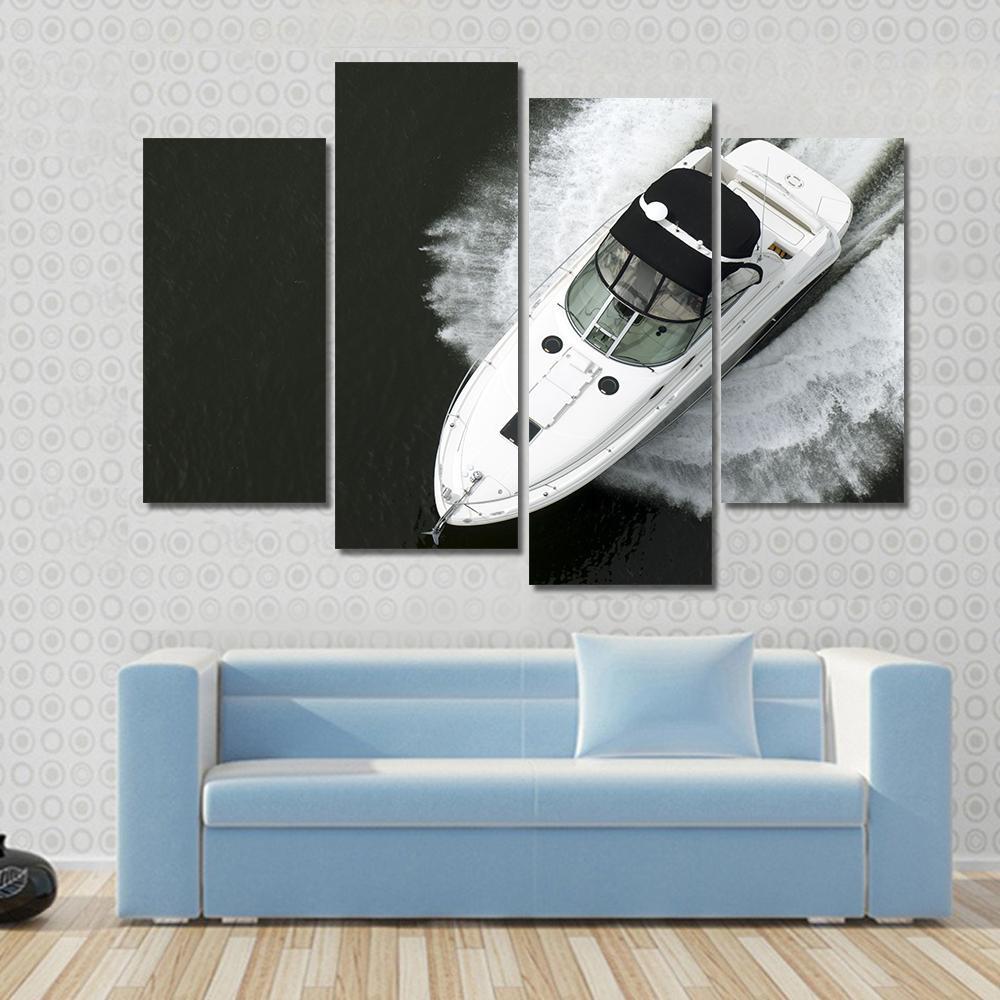The image depicts an impeccably staged, possibly digital, living room with a central pale blue couch adorned with a matching single cushion. The room exudes a minimalist elegance, emphasized by a light wooden plank floor and a back wall draped in sophisticated grayish-silver wallpaper embellished with various circular patterns. Dominating the wall behind the couch, there is a striking black and white nautical scene spread across four vertically aligned rectangular panels. These panels collectively form a cohesive image of a yacht gliding through the water, with the inner two panels being slightly larger than the outer ones. This art piece, along with the clean and modern furnishings, suggests that the setting is an idealized illustration, potentially created with Photoshop for use in a home décor website. Off to the right side of the couch on the floor, one might notice a mysterious black object, adding a subtle touch of intrigue to the otherwise serene environment.